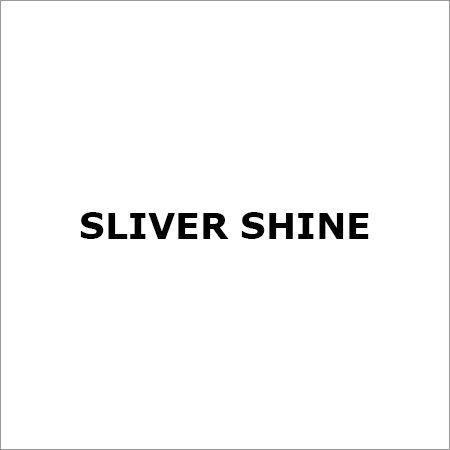The image is minimalistic and strikingly simple, featuring a solid white background framed by a very thin black border. At its heart, the image presents two small, bold, black words: "Sliver Shine," directly centered and surrounded by expansive white space. This centered text, reminiscent of a book's typography, emphasizes clarity and elegance. The overall effect is stark yet stylish, with the black text clearly standing out against the pristine white backdrop.